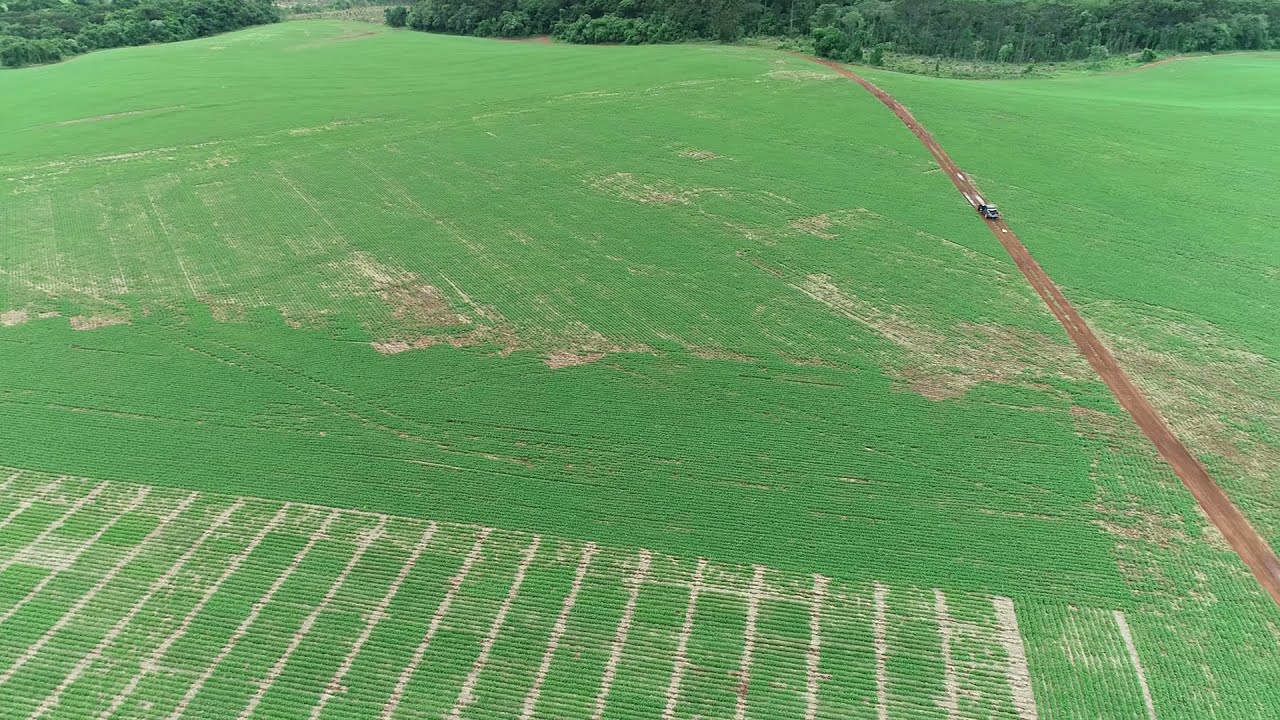The image captures an elevated view of a vibrant green farmland, segmented into neat, horizontal planting rows interspersed with earthy brown patches. A single-lane, reddish-orange dirt road runs diagonally from the bottom right corner towards the top left, bisecting the landscape. A truck is seen driving along this road. Along the top edge of the image, a line of trees forms a natural border, extending just beyond the frame. The camera, positioned approximately 100 feet above the ground, angle down slightly, provides a comprehensive view of this tranquil rural scene.